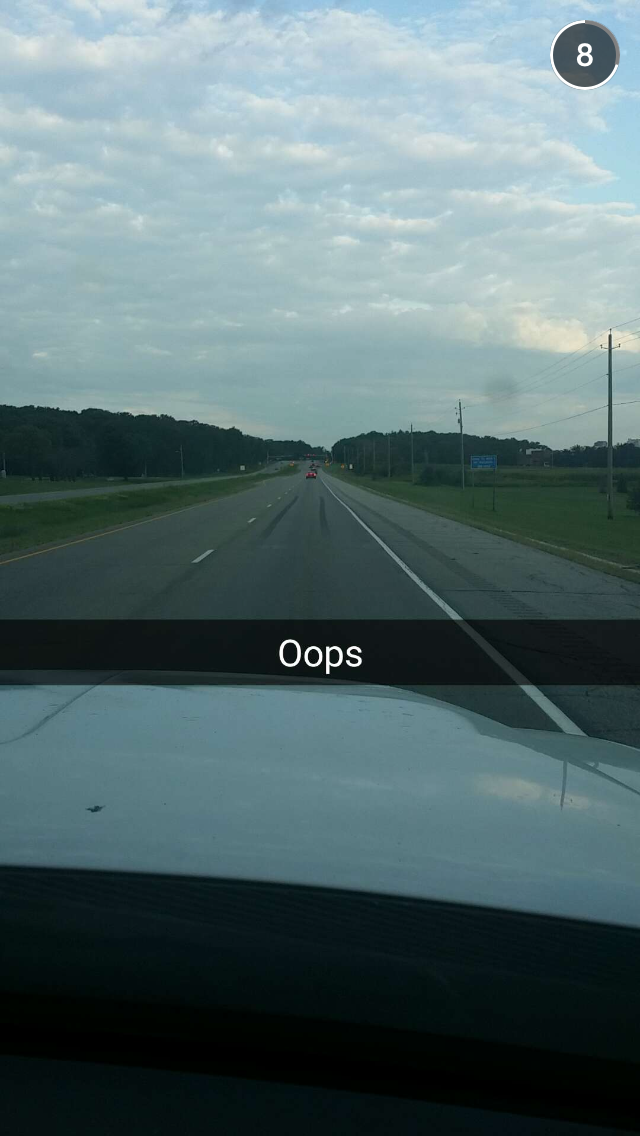A detailed caption for this image could be:

"Inside view from a vehicle on a two-lane interstate, possibly captured for Snapchat with a gray caption bar reading 'oops' positioned across the middle of the image. The interior of the vehicle isn't clearly visible, but the wide, white hood dominates the foreground. The driver navigates the outer lane as another vehicle far ahead displays its brake lights. Trees line the highway, stretching into the distance, with lush green grass in the median and along the roadside. Fluffy white clouds dot the partly cloudy sky, hinting at either early morning or late evening."